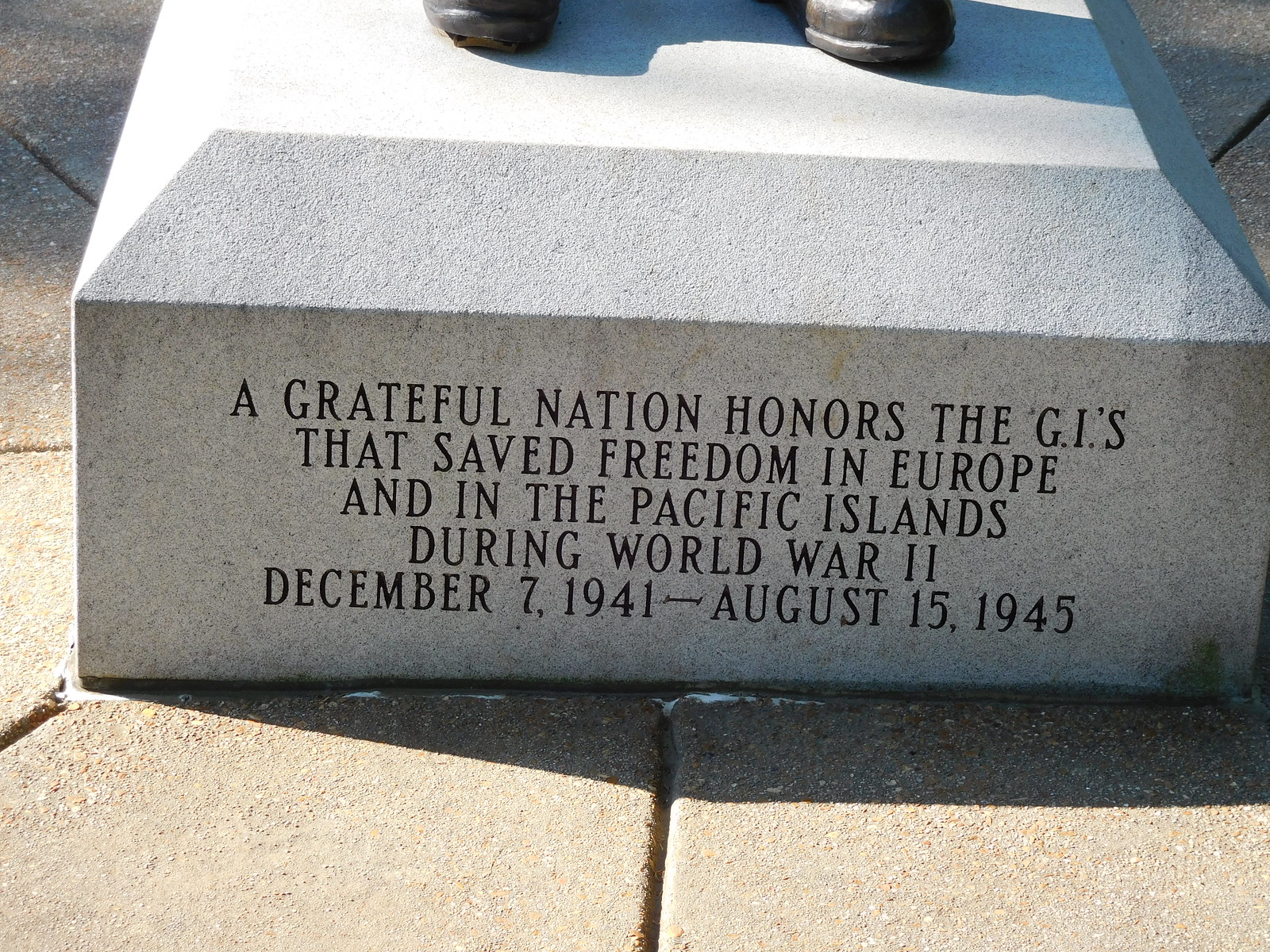The photograph displays the base of a monument or statue set outdoors on what appears to be a stone or concrete street. The base is a large, square, gray slab, possibly made of concrete, and features a prominent engraving that reads: "A grateful nation honors the G.I.s that saved freedom in Europe and in the Pacific Islands during World War II, December 7, 1941 to August 15, 1945." Only the very bottom of the statue is visible, revealing what seems to be the edges of metal or bronze shoes. The base has slightly inward-curving sides and is centered on what looks like a concrete pad with lines extending from it, suggesting a structured pavement design around the memorial.